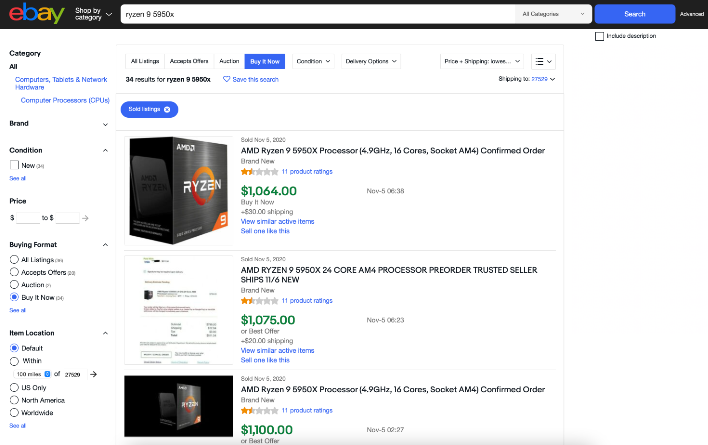This screenshot captures a user’s interaction with the eBay website, displayed in landscape mode. In the top left corner, the familiar eBay logo is prominently visible, followed by the option to "Shop by category." Just below, a search bar indicates the user has typed in "RYZEN 9 5900X." In the upper right corner, there's a prominent blue search button.

The search results reveal Ryzen products currently available for sale. The webpage layout features two main columns. The left-hand column presents several filtering options. It starts with broad categories such as "All," "Computers," "Tablets & Network Hardware," narrowing down to "Computer Processors (CPU)." Further filtering options include "Brand," "Condition" with a checkbox for "New" (which hasn't been selected), and a price range feature designated by dollar signs. The user has specifically chosen the "Buy It Now" format, indicating their preference to purchase immediately rather than via auction or accepting offers.

Additionally, the item location filter remains at the default setting, which typically limits the search to items available within a certain proximity, possibly within 100 miles. 

On the right side of the page, the relevant "Buy It Now" listings for AMD Ryzen 9 5900X are displayed, with prices ranging from $1,064 to $1,100. The user's final decision might hinge on the associated shipping costs for these items.